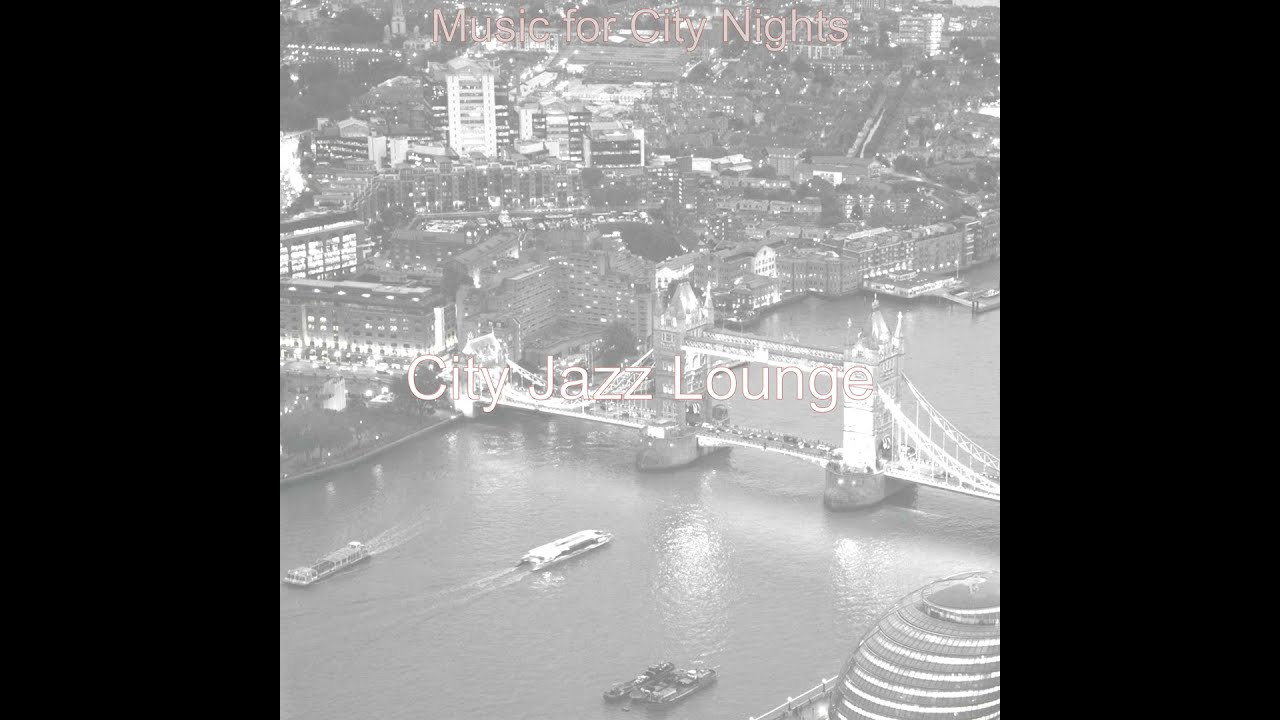The image captures a high-angle, nighttime cityscape, predominantly in black and white. The scene is framed by two vertical black bars on the left and right sides. Up top, tiny red text reads "Music for City Nights." Below, the text "City Jazz Lounge" appears in white across the center. The central feature is a large suspension bridge stretching across a waterway. Multiple boats navigate the water, with some sailing towards the viewer and others away. The densely packed city in the background is illuminated by twinkling lights from various buildings, adding to the bustling, vibrant atmosphere. The overall hazy, faint coloring gives a slightly fuzzy appearance to the image, enhancing its dreamy, artistic quality.